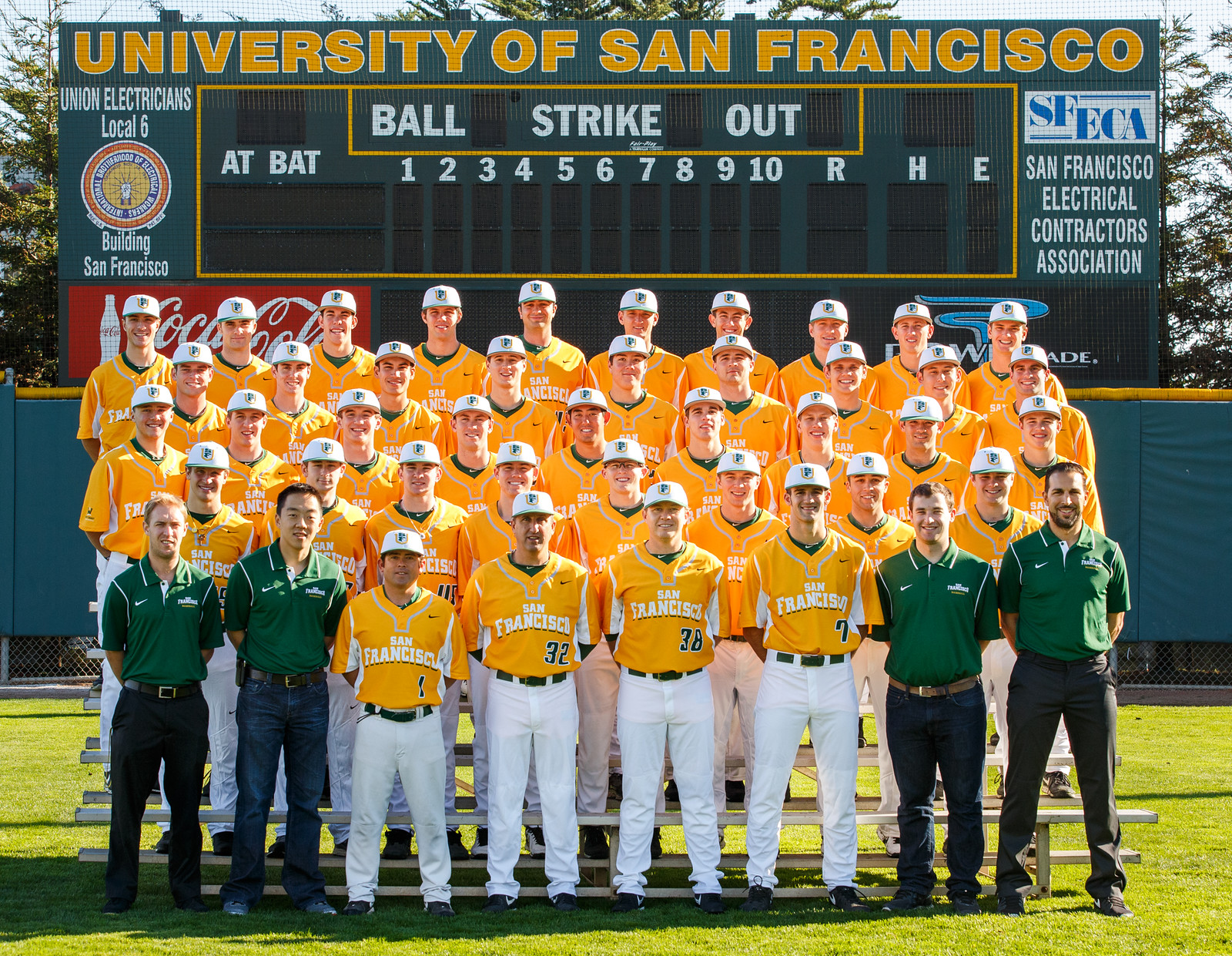In this vibrant, sunny photograph, the University of San Francisco baseball team is assembled for a team picture on a lush green field, likely part of their home baseball stadium. The team is organized in five distinct rows, with players and managers systematically positioned on a series of risers, ensuring every member is clearly visible. The players are attired in bright marigold yellow shirts paired with white pants and dark belts, while the two referees standing at either end of the front row sport dark green polo shirts and black slacks.

Dominating the background is a large, green scoreboard adorned with orange lettering spelling out "University of San Francisco." The scoreboard prominently features essential game categories such as Ball, Strike, Out, At Bat, Innings, Runs, Hits, and Errors. Advertisements for Union Electricians Local 6 and the San Francisco Electrical Contractors Association (SFECA) flank the central scoreboard. Additionally, a notable Coca-Cola sign is visible at the bottom alongside a Powerade logo.

The team stands in front of green padding on the fence, with the bright sunlight casting a warm glow across the scene, further emphasizing the team's vivid attire and the well-maintained grass of the field.